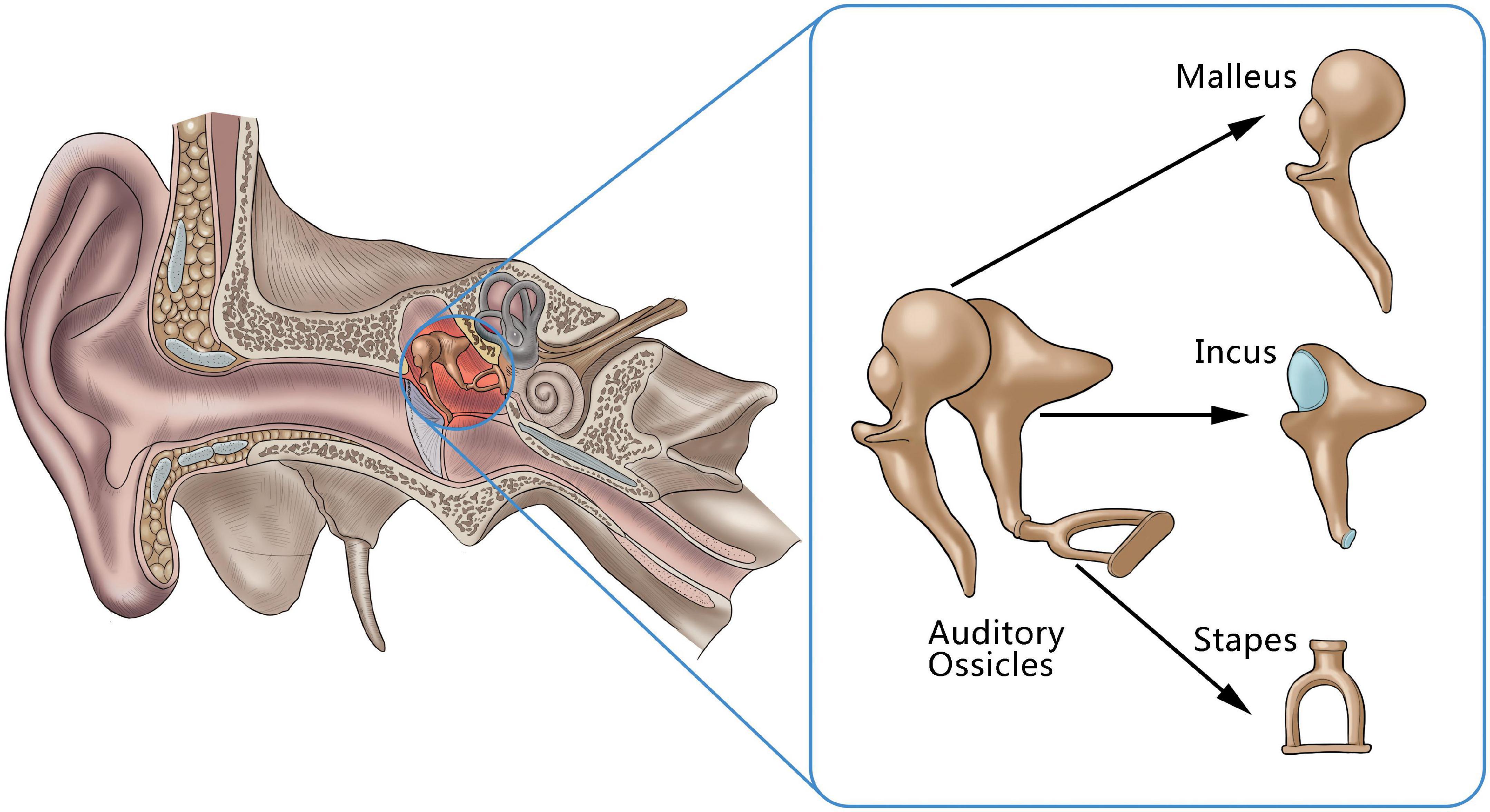The image is a detailed color diagram of the human ear, prominently displaying its inner structure. On the left side of the diagram, a rendering presents an external view of the ear, showing the outer ear, the ear canal, and how the canal connects to the inner ear within the human head. The ear canal is depicted in a pinkish color, surrounded by beige illustrations of various anatomical parts and canals. A blue circle highlights the middle ear bones, which are shown more prominently in a blue box on the right side of the image.

This blue box on the right magnifies and labels the middle ear bones—the malleus, incus, and stapes—detailing each one individually. The malleus is characterized by a round top connected to a stick-like handle. The incus is depicted with a hollow area, and the stapes is represented by a shape resembling a hammer with a handle. Together, these bones form the auditory ossicles, crucial for hearing, and their detailed renderings offer a clearer understanding of their shapes and interactions within the ear. The diagram as a whole provides an informative visual of both the collective and individual structures of the middle ear bones against a clean white background.